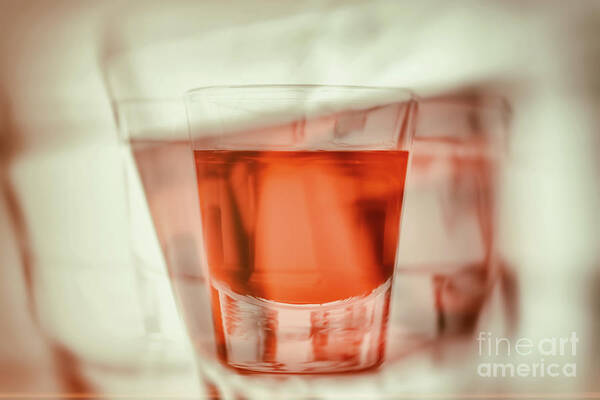The image showcases an artistic photograph of a transparent shot glass with a thick base, centrally positioned against a white-greenish background. The shot glass contains a reddish-orange liquid, possibly suggesting an alcoholic beverage or cocktail. Overlapping projections and diffused reflections create a complex, layered effect, with hues of reddish-orange spilling onto the backdrop, which resembles a folded or slightly textured canvas. The top of the glass is not completely filled, adding to the focus and depth of the composition. A subtle pinkish tint edges the background, reinforcing the overall theme of glassware and alcoholic drinks. The bottom right corner of the image reveals the white text "Fine Art America," signifying its stylistic inclination towards fine art photography.